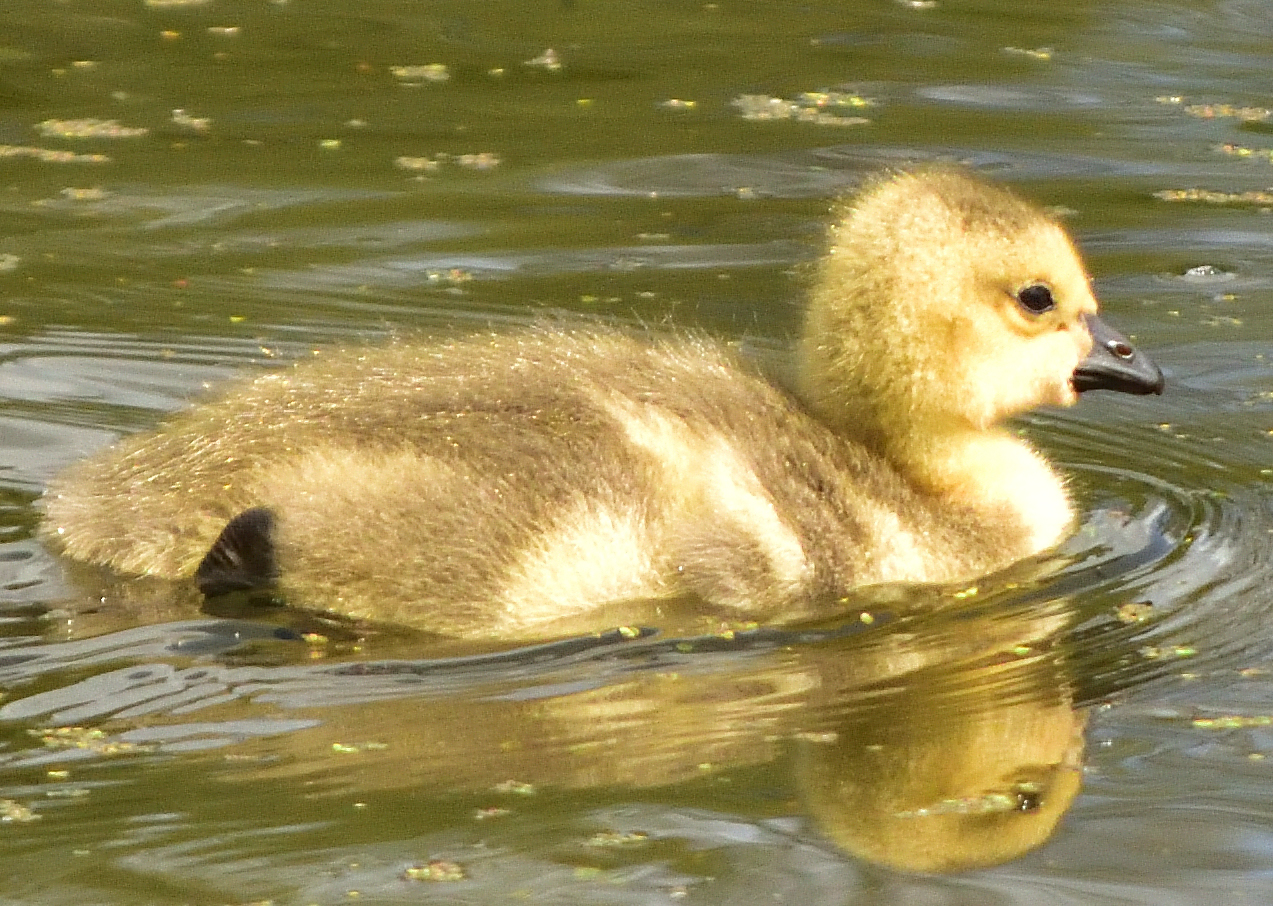This nature photograph captures a close-up of a yellow and brown baby duckling, also known as a duckling, swimming in a calm, greenish pond. The duckling is positioned in the center of the image, showing its profile with its black beak pointed to the right. The adorable creature has fuzzy, yellow and dark brown feathers with a striking black eye, and its little feet are hidden beneath the water's surface. Surrounding the duckling are floating bits of plant matter, including green leaves and algae, adding texture to the serene, rippling water. The reflection of the duckling in the water enhances the tranquil ambiance of the setting.